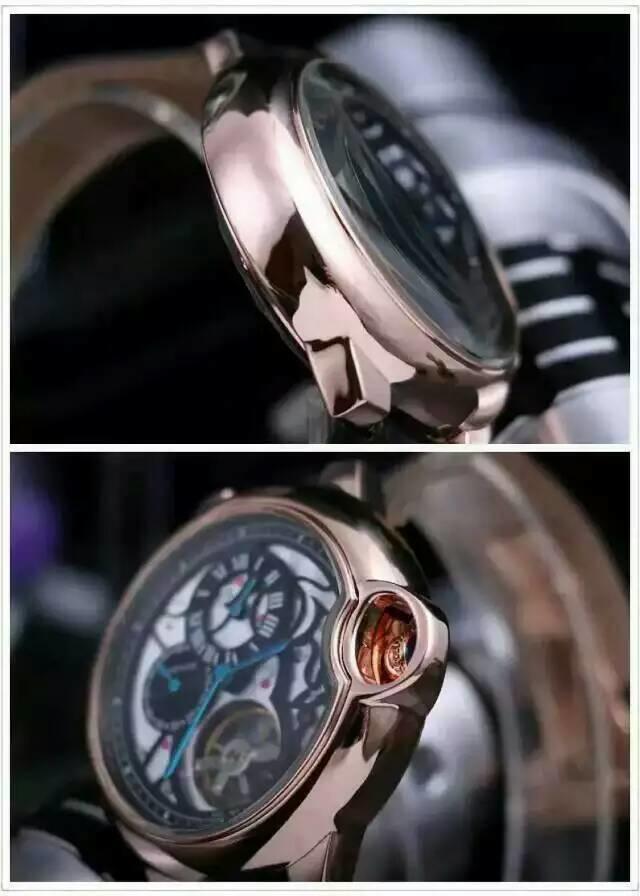This composite image consists of two pictures of a wristwatch, separated by a white line. The top image showcases the watch turned to its right side, highlighting its metallic face and brown band. Situated to the right of the watch is an indistinct white object. The bottom image presents the same watch, but from an alternate angle, with the watch face now oriented to the left. This perspective allows for a clearer view of the watch's face, revealing three smaller round sub-dials embedded within it.